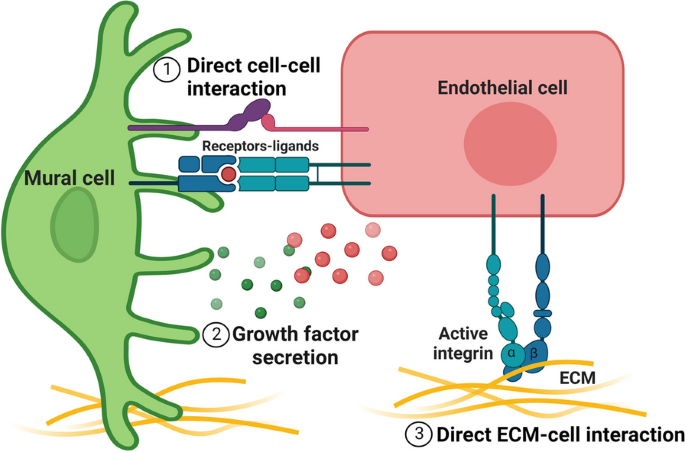The image depicts a detailed biological diagram on a white background featuring a complex cell interaction process with multicolored elements and textual annotations. On the left side, there is a green complex structure resembling an octopus, labeled "mural cell," characterized by several arm-like extensions and a notable circle. Adjacent to this is a black circled number labeled "1" indicating "direct cell-to-cell interaction." Next, a pink rectangle on the right side, containing a darker pink circle, is labeled "endothelial cell." Between the mural cell and endothelial cell, various elements highlight key biological pathways: "2" indicates "growth factor secretion," represented by green and pink dots merging, and "3" points to "direct ECM-cell interaction," involving blue components labeled "active integrin" and "ECM." The diagram includes blue rectangles connected by black and green lines, with a red dot in the center marked "receptors" and "ligands," illustrating the interplay between these cellular and molecular structures.